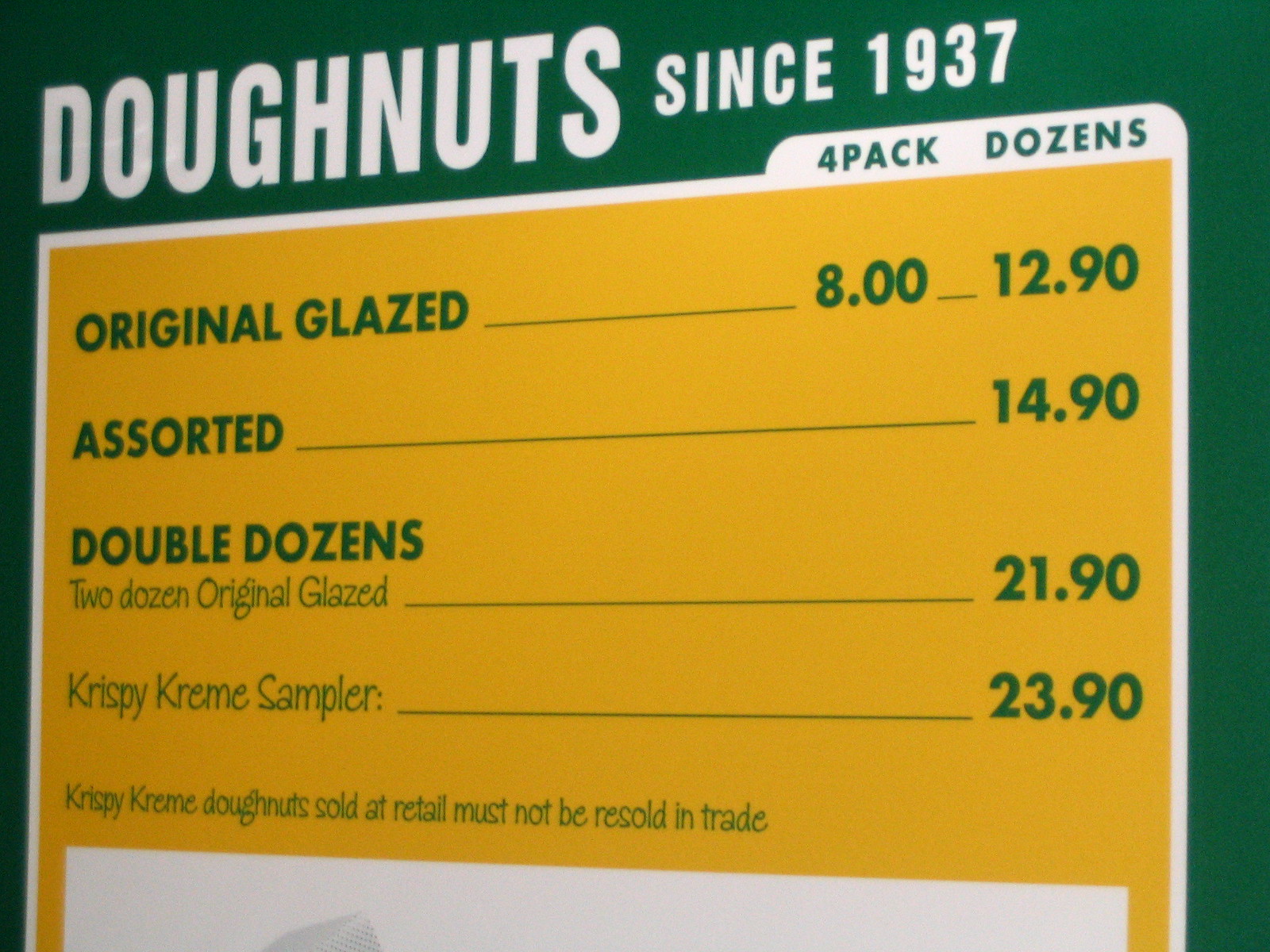The image showcases a detailed, horizontal rectangular menu board from a Krispy Kreme donut store. The menu board has a green background with prominent white text at the top reading "Donuts" and "Since 1937" below it in smaller letters. The central section of the board is yellow, featuring green text that lists various types of donuts and their prices. On the left side, the menu lists several donut options: "Original Glazed" in dark green lettering, priced at $8 for a 4-pack and $12.90 for a dozen; "Assorted" available for $14.90 per dozen; "Double Dozens" offering two dozen Original Glazed for $21.90; and the "Krispy Kreme Sampler" for $23.90. All the prices are clearly aligned on the right side. At the bottom of the menu, in smaller text, it states, "Krispy Kreme donuts sold at retail must not be resold in trade." The menu board is highly detailed and takes up the entire image frame, ensuring no other objects or background elements are visible, providing an in-store feel of viewing a real Krispy Kreme menu.